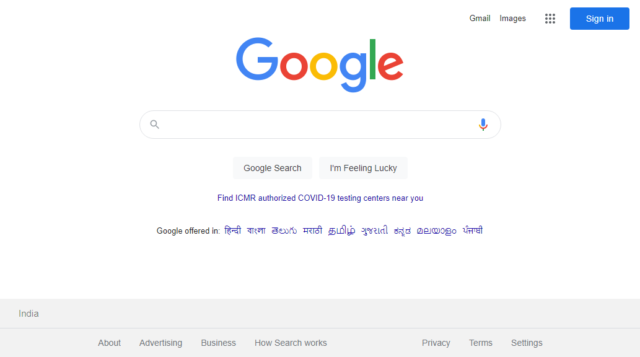The image is a screenshot of the Google search homepage. The background is predominantly white, with several elements arranged systematically. In the upper right corner, there are links in black font that read "Gmail" and "Images." Next to these links, there is an array of nine black circles arranged in a 3x3 grid. To the right of this grid is a blue button with white text that says "Sign In."

Centrally positioned on the page is the large and iconic Google logo, displayed in its usual multicolor scheme: a blue "G," a red "o," a yellow "o," a blue "g," a green "l," and a red "e." Below the logo is an empty search field, flanked on the right by a blue microphone icon and on the left by a gray magnifying glass icon.

Beneath the search field are two gray buttons: the left one labeled "Google Search" and the right one labeled "I'm Feeling Lucky." Lower on the page, there is a line of blue text that reads, "Find ISMR Authorized COVID-19 Centers Near You."

Further down, the text "Google offered in:" appears, followed by a list of languages written in Asian scripts, possibly including Hindi or another Indic language. Finally, at the very bottom of the page, a gray rectangle contains the word "India."